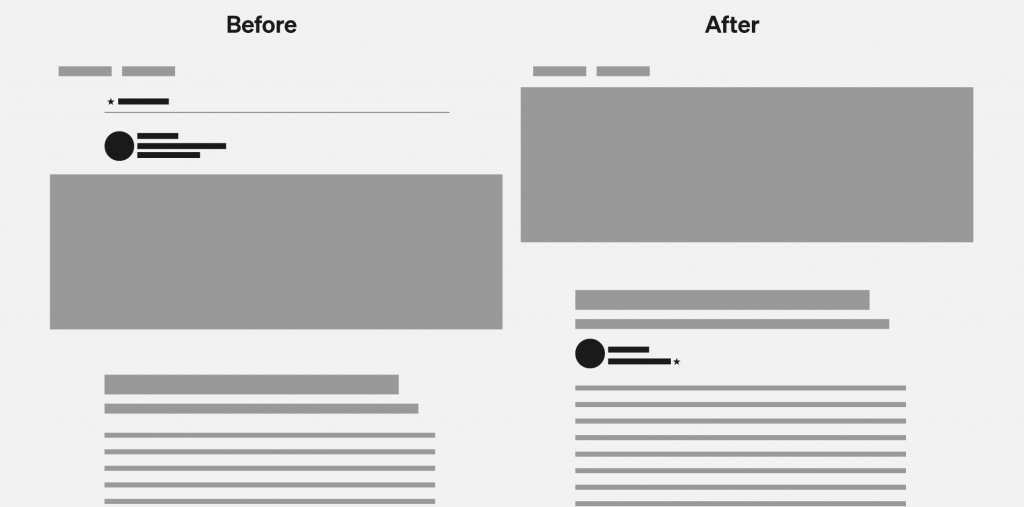The image presents a comparative side-by-side layout of a document labeled "Before" and "After." The original "Before" version features a plain document with several elements: a cluster of items at the top, a central banner, and a body of text below. This layout is designed to resemble a form with sections that look like redactions, though they are purely illustrative to showcase the page layout. 

In the "After" version, the layout has been significantly reorganized. The elements that were initially at the top have been relocated to below the central banner, resulting in the majority of the text now appearing beneath the banner. This highlights a shift in the arrangement of paragraphs, titles, and other textual elements on the page.

The background color of the document is a soft light gray, while the text and layout elements are depicted in a darker gray. There is also a prominent black section, which appears to be designated for critical information such as the recipient's or sender's name.

Overall, the image serves as a visual representation of how different document elements can be arranged on a page, emphasizing the subjective nature of layout preferences.